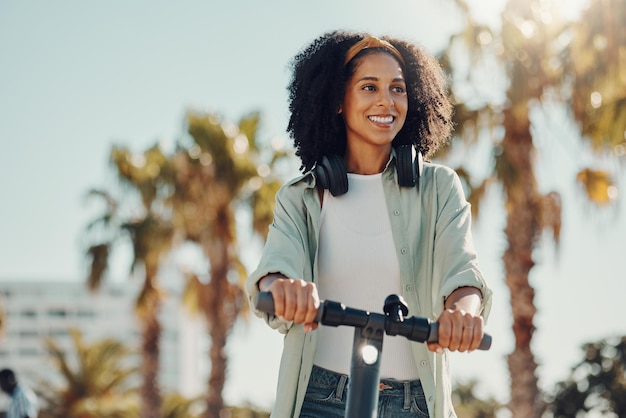In this vibrant outdoor scene, a young black woman with shoulder-length curly hair, adorned with a bandana and sporting large headphones around her neck, stands confidently on an electric scooter. She is radiating a joyful smile, dressed casually in a green shirt, a white undershirt, and blue jeans. The scooter is equipped with a light, highlighting its modern, sleek design. It’s a sunny, tropical day, suggesting a warm climate, possibly in Miami. The background features an array of lush palm trees and a white building, adding to the tropical ambiance. The bright sunlight bathes the scene in light greens and yellows, capturing a lively, cheerful mood. Amidst this, other elements, such as a blurred pedestrian and hotel, contribute to the dynamic urban setting.